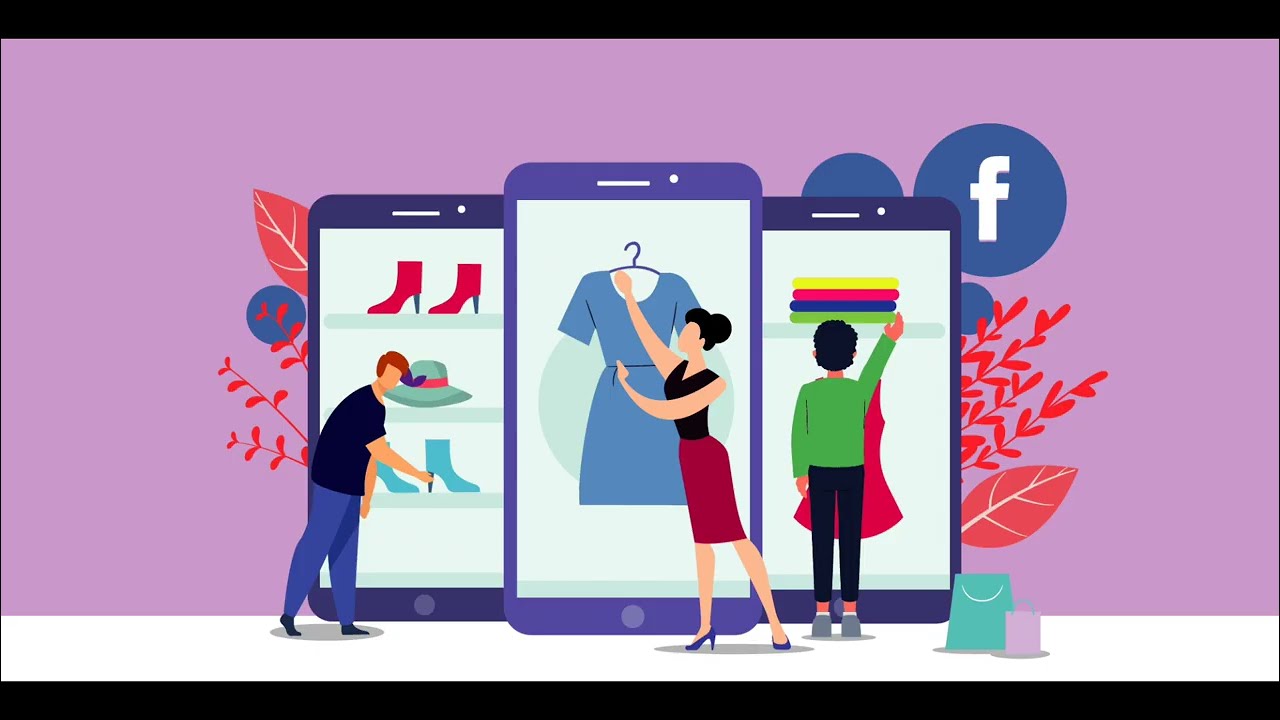The image portrays a digitally illustrated scene, likely from an instructional or tutorial video, with a lavender background and a white floor. Central to the composition are three towering cell phones that stand taller than the people depicted with them. The overall artwork style features faceless, shapeless characters in a corporate, minimalist design. 

Occupying the middle cell phone is a purple-outlined screen displaying a blue dress. A woman with a black blouse, red skirt, and a bun stands in front of it, seemingly adjusting the dress. The left cell phone showcases shelves with high-heeled boots and a hat, while a man in a dark blue shirt and pants gestures towards a boot. The right cell phone displays folded clothing on shelves and a red dress, with a person in black pants and a green shirt, viewed from behind, pointing at the items. 

In the top right corner of the image, the Facebook logo, a white lowercase "f" in a blue circle, is visible. Outlines of red decorative plants and leaves frame the sides of the cell phones. On the floor, near the rightmost cell phone, are a few shopping bags, adding to the commercial theme. The overall impression is one of a modern, corporate digital illustration, possibly used in an advertisement for Facebook clothing or fashion-related content.